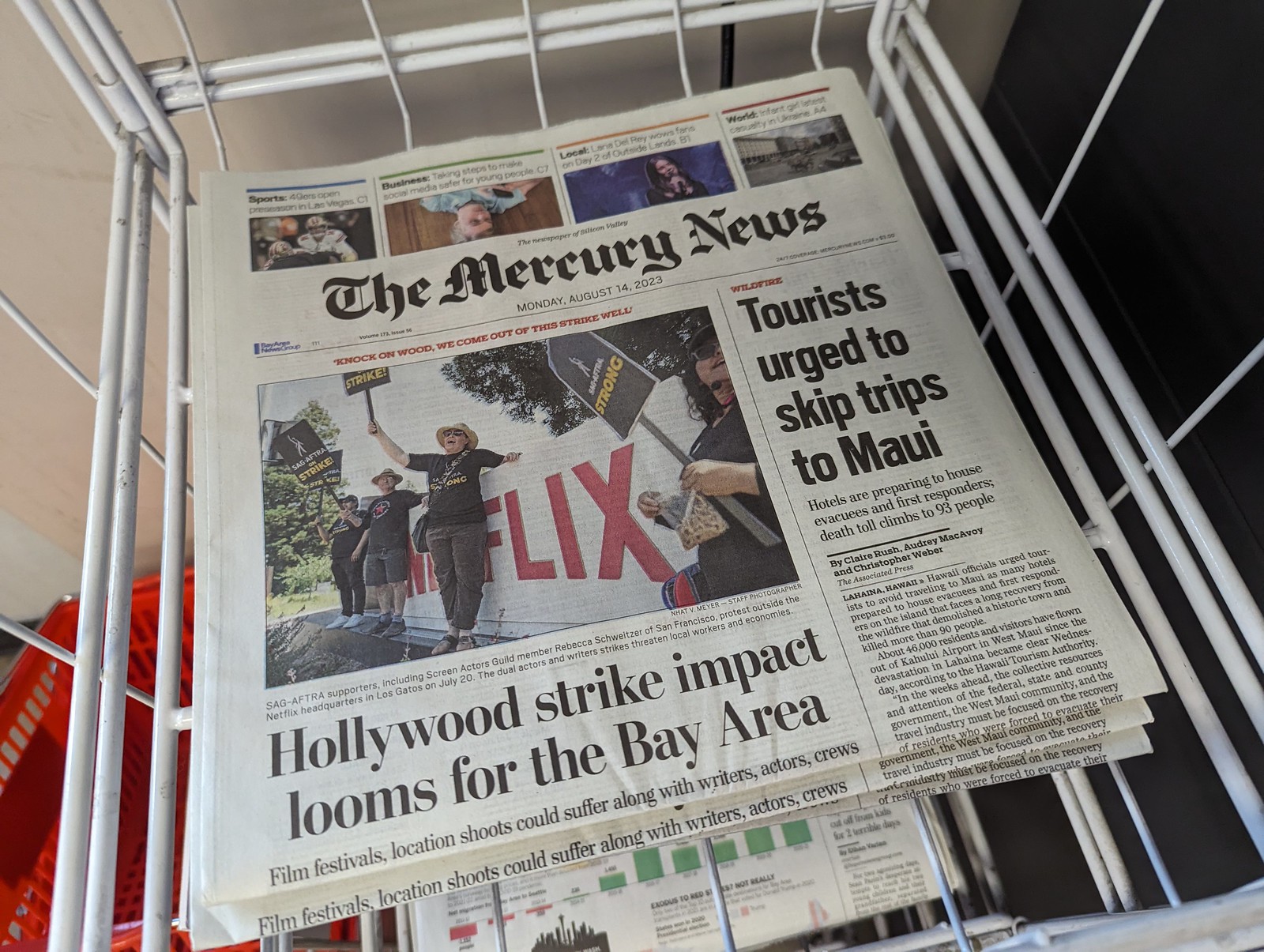The front page of the Mercury News, dated Monday, August 14, 2023, is prominently displayed on the top shelf of a white wire bin within a public display rack. The dominant feature is a large, colorful image of numerous people picketing in front of the Netflix sign, all dressed in black shirts and holding black signs with yellow lettering that reads "WGA Strong" in support of the Writers Guild strike. The headline below this image reads, "Hollywood Strike Impact Looms for the Bay Area." To the right, another significant story headline states, "Tourists Urged to Skip Trips to Maui." Above the newspaper's masthead, there is a small bar featuring four different photographs, each with its own story headline. In the background is a grayish-tan color, and a small orange shopping basket with a silver handle appears in the bottom left corner of the image.